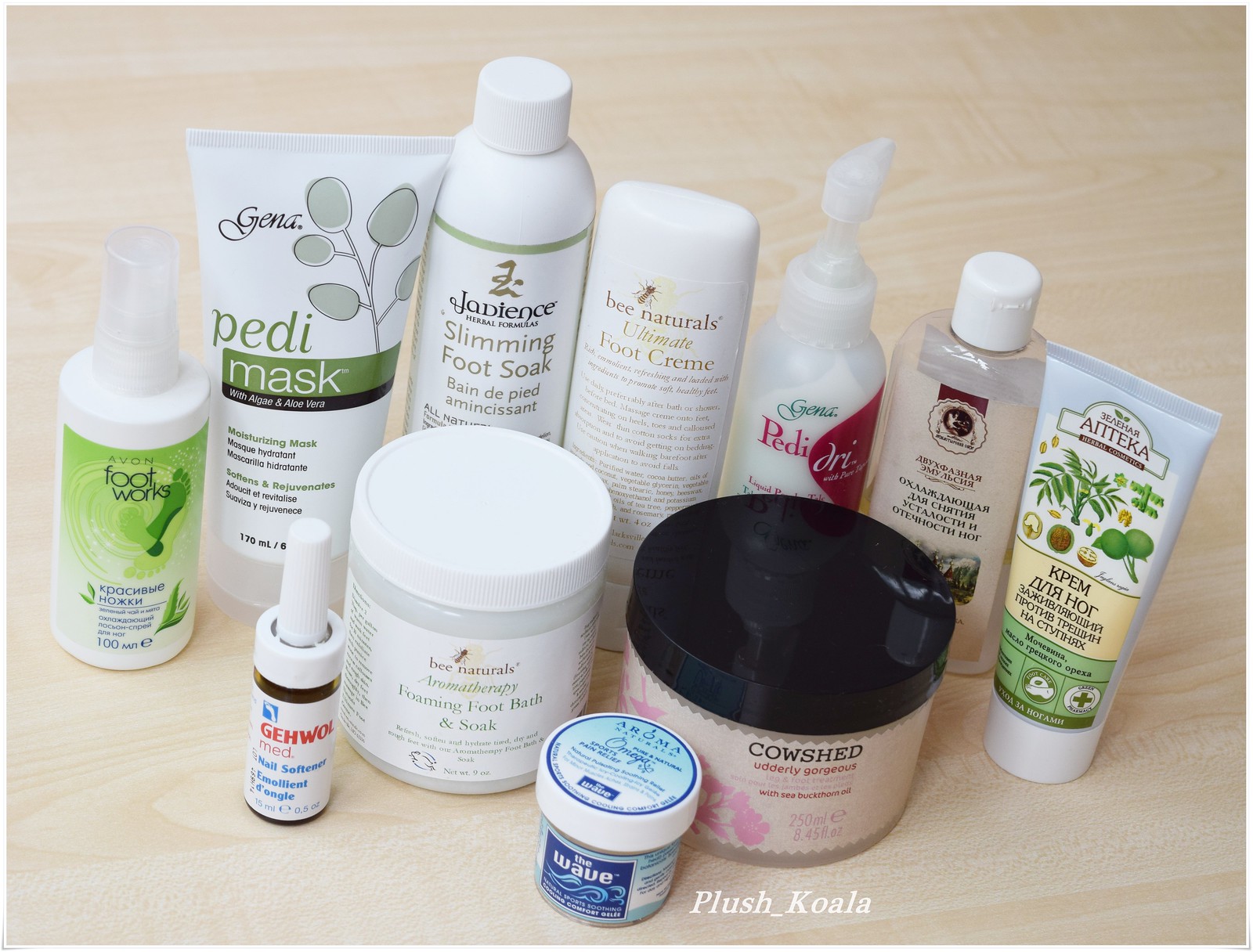A meticulously arranged display of cosmetics and skincare essentials adorns a creamy off-white background, stretching diagonally from the top left to the bottom right. The ensemble features a thoughtfully staged assortment of jars, tubes, and pump bottles. The items are strategically placed akin to a school group photograph, with height gradients peaking in the center and tapering towards the edges.

In the back row, seven bottles and tubes stand tall, showcasing a variety of sleek and elegant packaging. Dominating the foreground are two substantial round jars—one pristine white with a matching lid on the left, and a chic pink jar paired with a contrasting black lid on the right. Nestled in front of these jars, to the left, is a white medicinal bottle crowned by a protruding rubber stopper, hinting at an enclosed eye dropper.

Positioned slightly in front of the lower half of the pink jar is a smaller, vibrant blue jar. It proudly features a blue label inscribed with the word "WAVE" in bold white letters. Adjacent to this, the words "PLUSH KOALA" stand out in white, emblazoned against the soft background, adding a playful yet sophisticated touch to the arrangement.